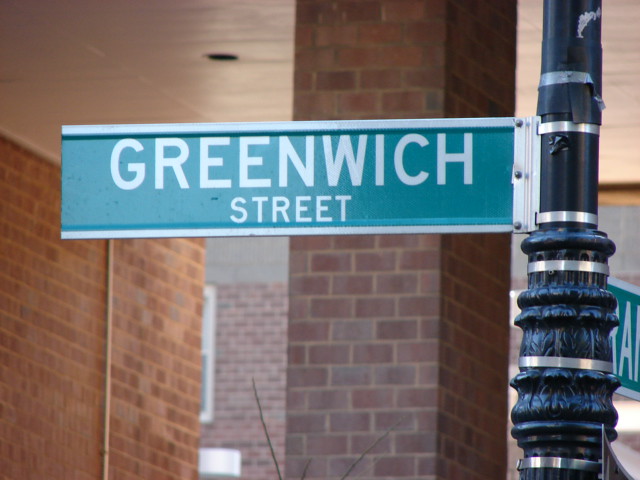In the photograph, a striking street sign is prominently displayed, set against the backdrop of a red brick building. The signpost is an exquisite piece of craftsmanship made of black wrought iron, adorned with intricate, ornate patterns and bands of silver that catch the light. The street sign itself contrasts with this historical elegance, being a modern-style green sign with white lettering that reads "Greenwich Street." The word "Greenwich" is spelled out fully in white, clear capital letters, while "Street" is completely spelled out, which is atypical for American street signs. This detail raises curiosity about the location, suggesting that it might be a street sign found in England rather than the United States, where such street sign conventions differ. The juxtaposition of contemporary signage with the classical design of the pole makes this scene particularly captivating.